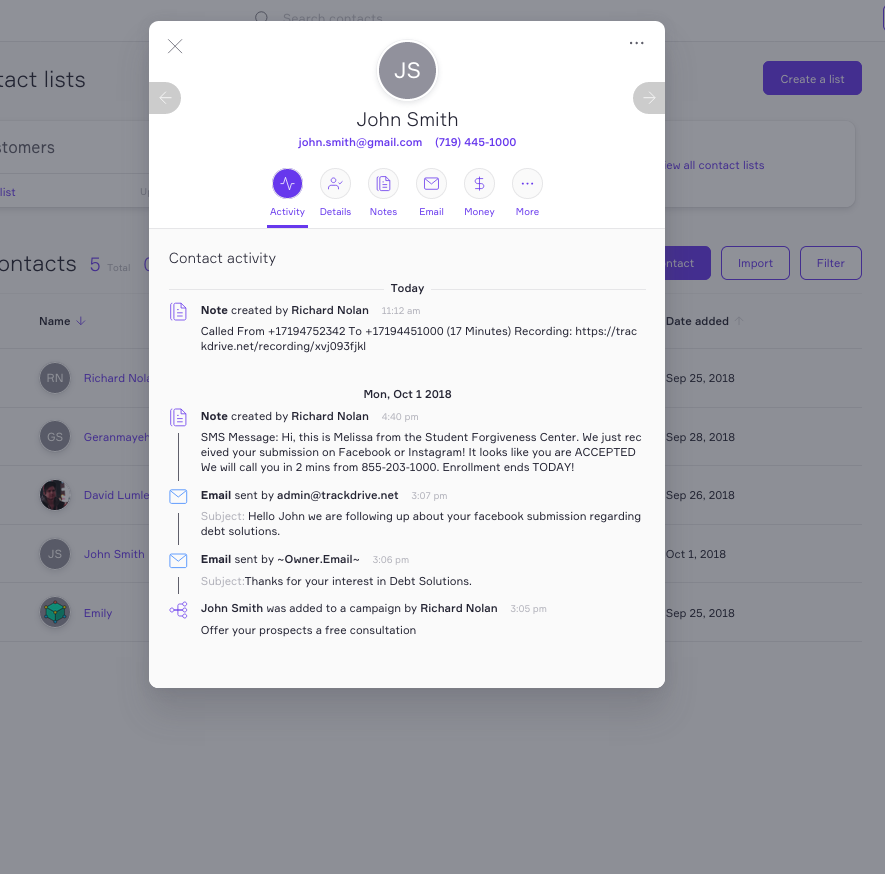The background of the image features a gray rectangle, largely obscured by an overlapping white rectangle in the foreground. The portion of the gray rectangle visible on the upper right side includes a purple box labeled "Create a List" and a purple-outlined rectangle below it labeled "Import," followed by another purple-outlined rectangle that says "Filter."

The white rectangle in the foreground has an "X" in the upper left corner for closing and three dots in the upper right corner, likely indicating more options. Below these, there is a gray circle with the initials "JS," under which the name "John Smith" is displayed, accompanied by an email address and a phone number. To the right of John Smith's details, there is a purple circle labeled "Activity" with a purple underline. Adjacent to this is a gray-outlined circle featuring a person icon, next to which is the word "Details." Following that are additional gray-outlined icons: a rectangle with purple paper labeled "Notes," a circle with a purple envelope labeled "Email," a circle with a dollar sign labeled "Money," and a circle with dots labeled "More."

Below these sections, the text "Contact Activity" appears, followed by a horizontal line, the word "Today," another horizontal line, and then several entries. The first entry includes a purple notes symbol with some unreadable words next to it and more text underneath. Another entry is marked "Monday, October 1, 2018," again with a notes symbol and subsequent entries connected vertically with lines. These lines lead to blue mail symbols and another indistinguishable purple symbol, with further descriptions in black text aligning to the left of these visuals.